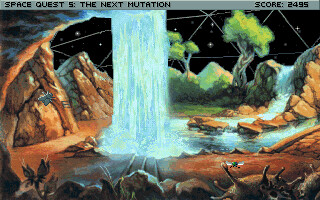The screenshot captured from the vintage video game "Space Quest V: The Next Mutation," showcases its charmingly simplistic and nostalgic graphics. Displayed within a basic, low-resolution format, the image exudes a quaint yet captivating appeal typical of classic video games. Dominating the scene is a picturesque waterfall cascading through an overhead portal into a serene, dreamlike pond dotted with boulders. The intricate environment includes fascinating stalactites and stalagmites, along with peculiar cave creatures and exotic cave flora positioned in the lower left corner. Trees can be seen in the distance, creating an illusion that the viewer is inside a fantastical, glass-enclosed biome. The distant crisscross pattern suggests we are viewing the scene from within a living sphere or dome, further enhancing the otherworldly experience. The upper silver-gray border displays the game title, "Space Quest V: The Next Mutation," and the player's score, 2455 out of 2495. The backdrop of stars visible through the dome completes the ethereal atmosphere of this enthralling vintage game.